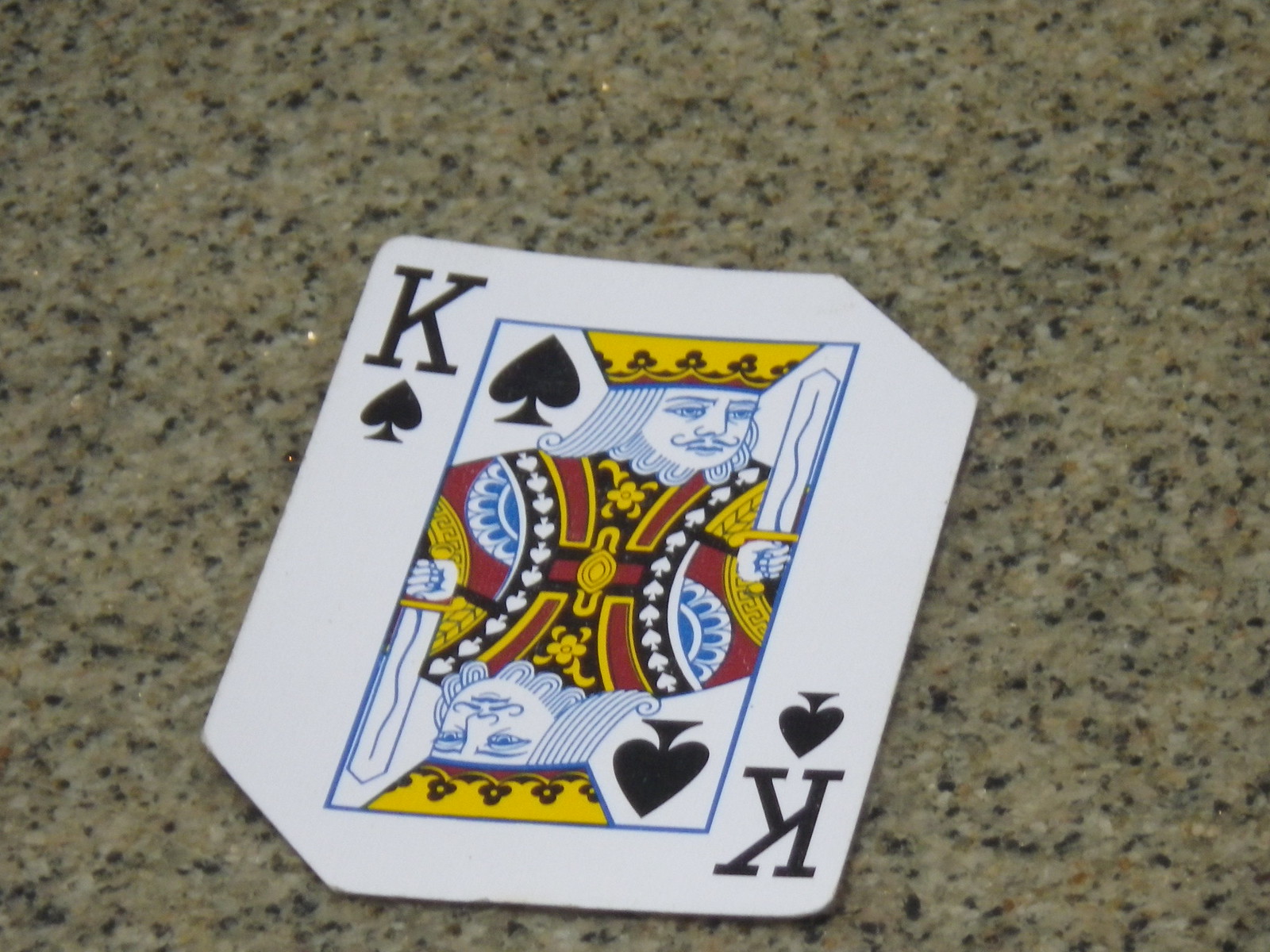The image showcases a distinctive King of Spades card that deviates from the standard playing card format. It is noticeably smaller with truncated corners—the upper right and lower left corners are cut off—giving it a non-traditional appearance. The card is displayed on a granite surface that features a complex pattern of black, cream, shades of gray, and off-white.

The artwork on the card depicts the King of Spades in a mirrored fashion; his upper body seamlessly transitions into his lower body, allowing him to be viewed right-side-up or upside-down. The King is dressed in a rich palette of gold, maroon, black, and white, and holds a sword prominently in both orientations. Each corner of the card contains a spade symbol inside a blue box: the upper left and lower right corners. Adjacent to these spade symbols, the letter 'K' is displayed, accompanied by a smaller spade symbol underneath. This unconventional playing card exudes an artistic and unique charm.